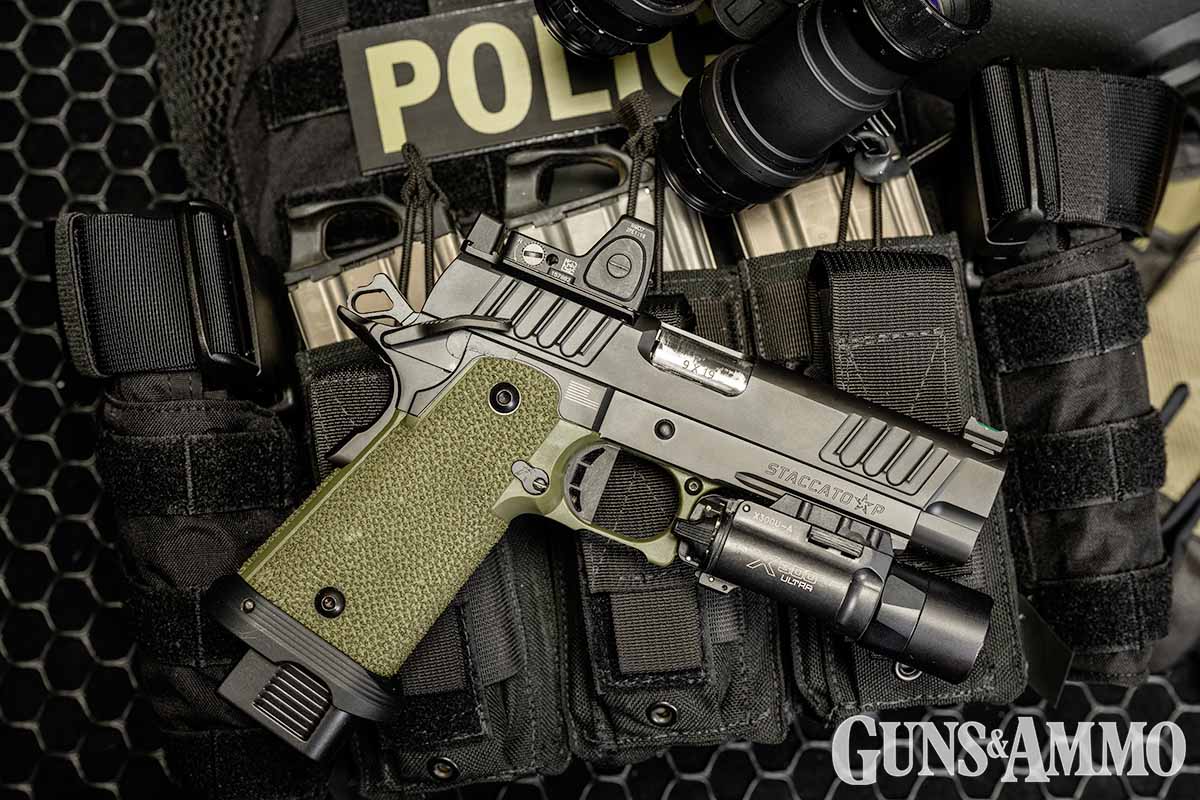This detailed aerial glimpse showcases a close-up of a police vest meticulously arranged with a handgun prominently displayed on top. The dark canvas and Velcro-laden vest clearly bears the word "POLICE," signifying its ownership. The firearm, a heavy-duty staccato P model, is equipped with an olive green textured grip and lies aiming towards the right. The magazine insertion point is visible at the bottom of the grip. Adding to the authenticity, the photo features a "Guns and Ammo" notation in the lower right corner, suggesting this image might be a professional product shot for a magazine or poster. The backdrop beneath the vest includes a black honeycomb grate, adding a contrasting texture to the overall composition.